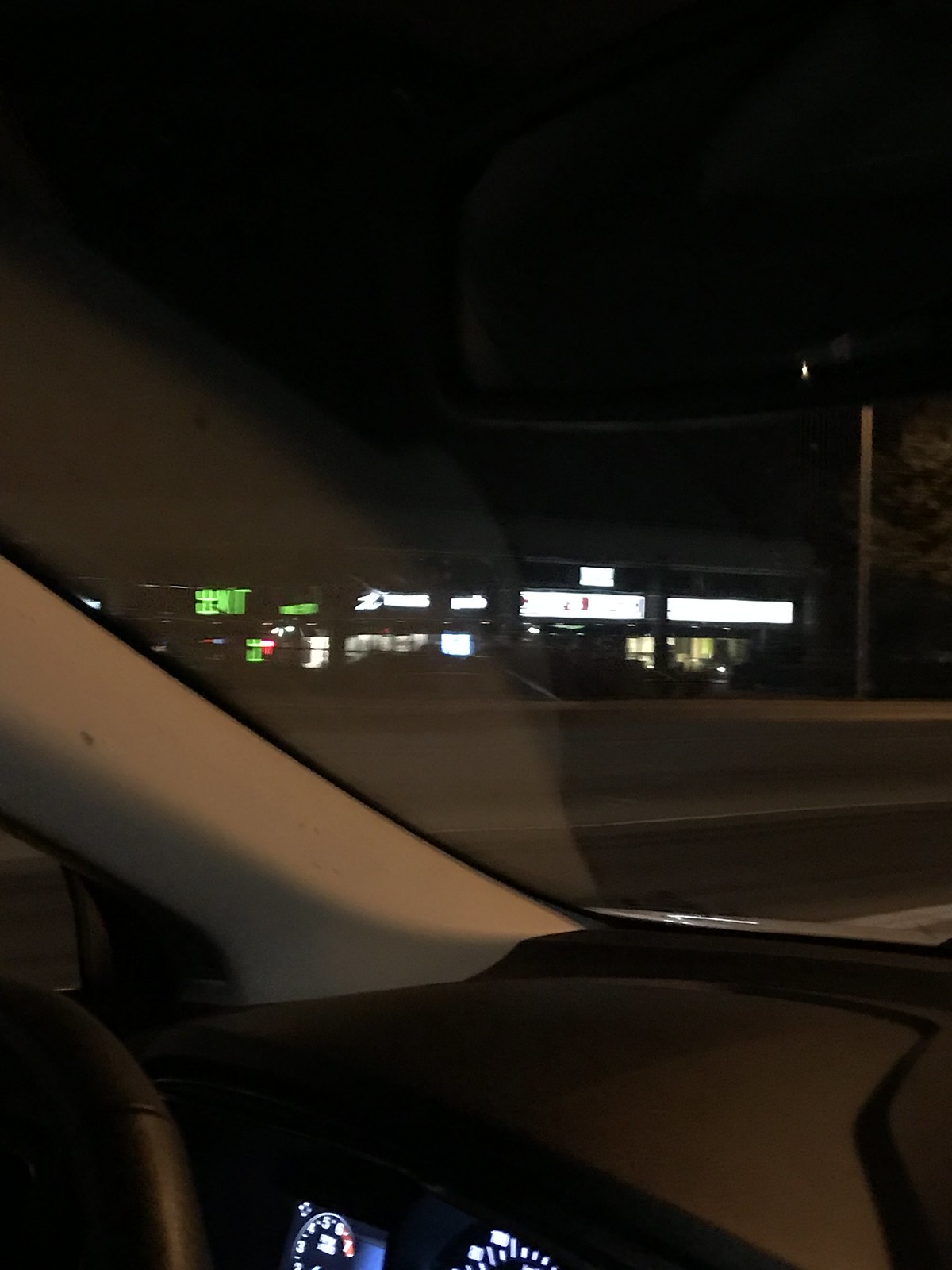This detailed photograph, taken in a portrait orientation from the passenger seat of a car, captures a multi-faceted scene. The car's interior is showcased prominently, with portions of the black steering wheel and dashboard in view. The windshield reveals a glimpse of the outside world, framed by the black fixtures of the car's interior. A unique contrast is provided by the white-colored segment leading up to the car’s roof. Through the windshield, a section of a street is visible along with a strip mall, which features several businesses illuminated by neon lights. The neon signs vary in color; the business on the far left is marked by a striking green light, while the others are adorned with vibrant white neon glow, adding a dynamic touch to the urban nightscape.